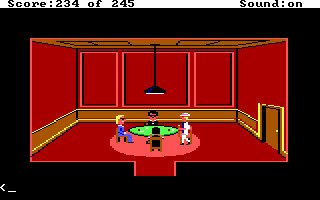A screenshot from a classic video game, likely from the 1980s or 1990s, depicts a vividly rendered indoor dining room. The setting features rich red hues dominating the tall ceiling and walls, which are adorned with red paneling and pink trim. A black light fixture hangs from above, casting an imagined glow over the scene. Central to the room is a round, green table, reminiscent of a poker table, around which several characters are seated, suggesting a social or gaming scenario. The characters — possibly male — vary in appearance with one sporting blonde hair, another with brunette, and a third with gray hair. The room's lower walls feature brown wainscoting accented with a yellow border, adding to the retro ambiance. To the right, a brown door with a visible handle hints at potential exits or entrances. Completing the scene, a score is displayed at the top of the screen, hinting at the game's competitive nature.